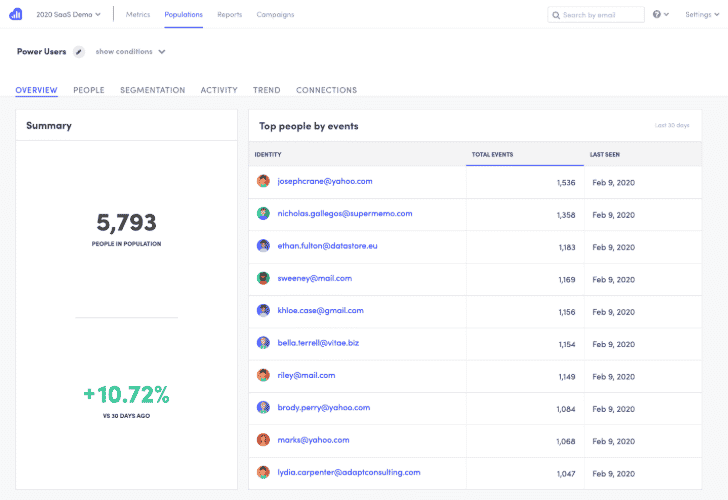In the image, we see a dashboard platform prominently labeled "2020 SAAS Demo" at the top, indicating a demonstration for a Software as a Service application. The interface features a navigation menu with four distinct tabs: Metrics, Populations, Reports, and Campaigns. Currently, the Populations tab is active.

Within the Populations tab, the screen is divided into two primary sections. On the left, there's an Overview section displaying a large number "5,793," representing the current population count. Below this figure, a percentage increase of "+10.72%" compared to 30 days ago is highlighted, indicating growth.

To the right of the Overview, there's a detailed list titled "Top People by Events." This section is organized into columns, including Email, Identity, Total Events, and Last Seen. Various user emails and event data are displayed, offering insights into the most active users based on their events.

Additionally, near the top of the screen, beneath the main navigation tabs, there is a section labeled "Power Users" with an edit button and a dropdown icon labeled "Show Conditions," providing functionality for further customization and filtering of data.

Overall, the interface provides a comprehensive view of user data and activity, allowing for in-depth analysis and monitoring of population metrics.